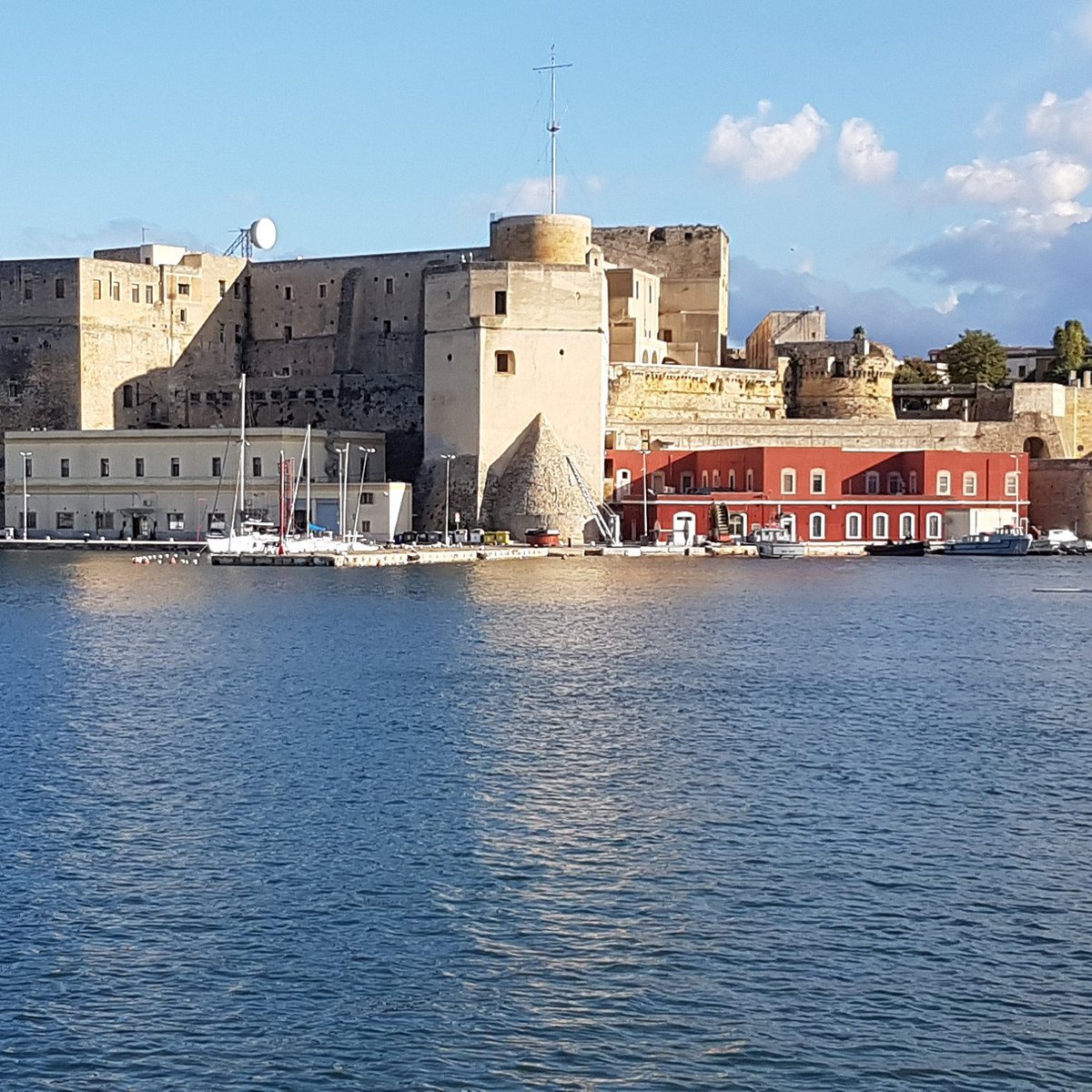A serene photograph captures a waterfront scene with calm, blue water in the foreground, reflecting an old-fashioned industrial complex along the shoreline. Central to the image, a large, square, stone-like building stands prominently, topped with a massive water barrel system and an electrical post resembling a cross. On the right side of this main building, a red brick, two-story factory with numerous windows is visible, surrounded by smaller tan and beige buildings of various shapes, including cylindrical and rectangular structures. To the left, a long, two-story factory building with rows of windows stretches out, featuring dark, wide docking bay doors at its base. Behind these structures, the largest building in the image, an L-shaped edifice that appears to be made of brick or stone, rises four or five stories high. This largest building also includes a satellite dish or similar fixture on its left top. Trees dot the background, emerging just below a light blue, partially cloudy sky. The water's edge hosts several docked sailboats and other vessels, suggesting a bustling port or dock area.